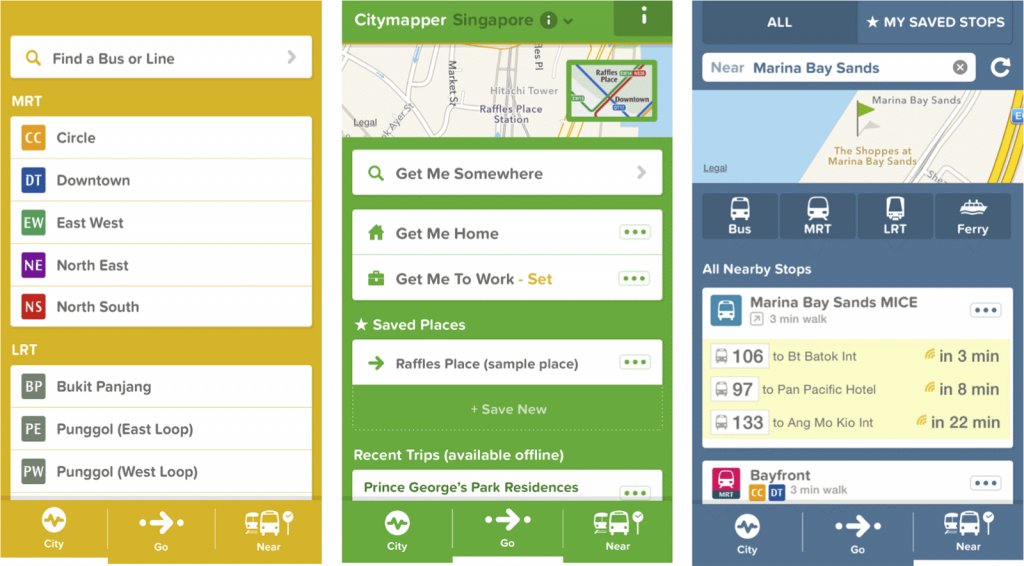These three screenshots from mobile devices display various public transportation apps with distinct visual designs and functionalities.

The first screenshot, on the left, features a mustard yellow background. At the top left, a white rectangular area with a golden magnifying glass icon contains the text "Find a bus or a line" followed by a gray arrowhead pointing right. Below this, bold, white capital letters read "MRT," listing options: Circle, Downtown, East-West, Northeast, and North-South lines. In another section, also in bold white capital letters, it says "LRT," with "BUKIT PANJANG," "PUNGGOL (East Loop)," and "PUNGGOL (West Loop)" listed consecutively.

The second screenshot, in the middle, displays a mossy green background. At the top left, the white rounded font spells "citymapper" with no space, followed by "Singapore" in dark green beneath it. To the right of this title, a dark green circle with a white lowercase "i" symbolizes additional information availability, followed by a downward-pointing arrowhead and a green square with another lowercase "i." Below this section, a small map is visible with a highlighted area enclosed within a green square border. Further down, a green background area states "Get me somewhere," with specific options labeled "Get me home," "Get me to work," and "Raffles Place (sample place)."

Together, these screenshots depict different sections and functionalities of mobile applications designed to aid users in navigating public transportation systems.